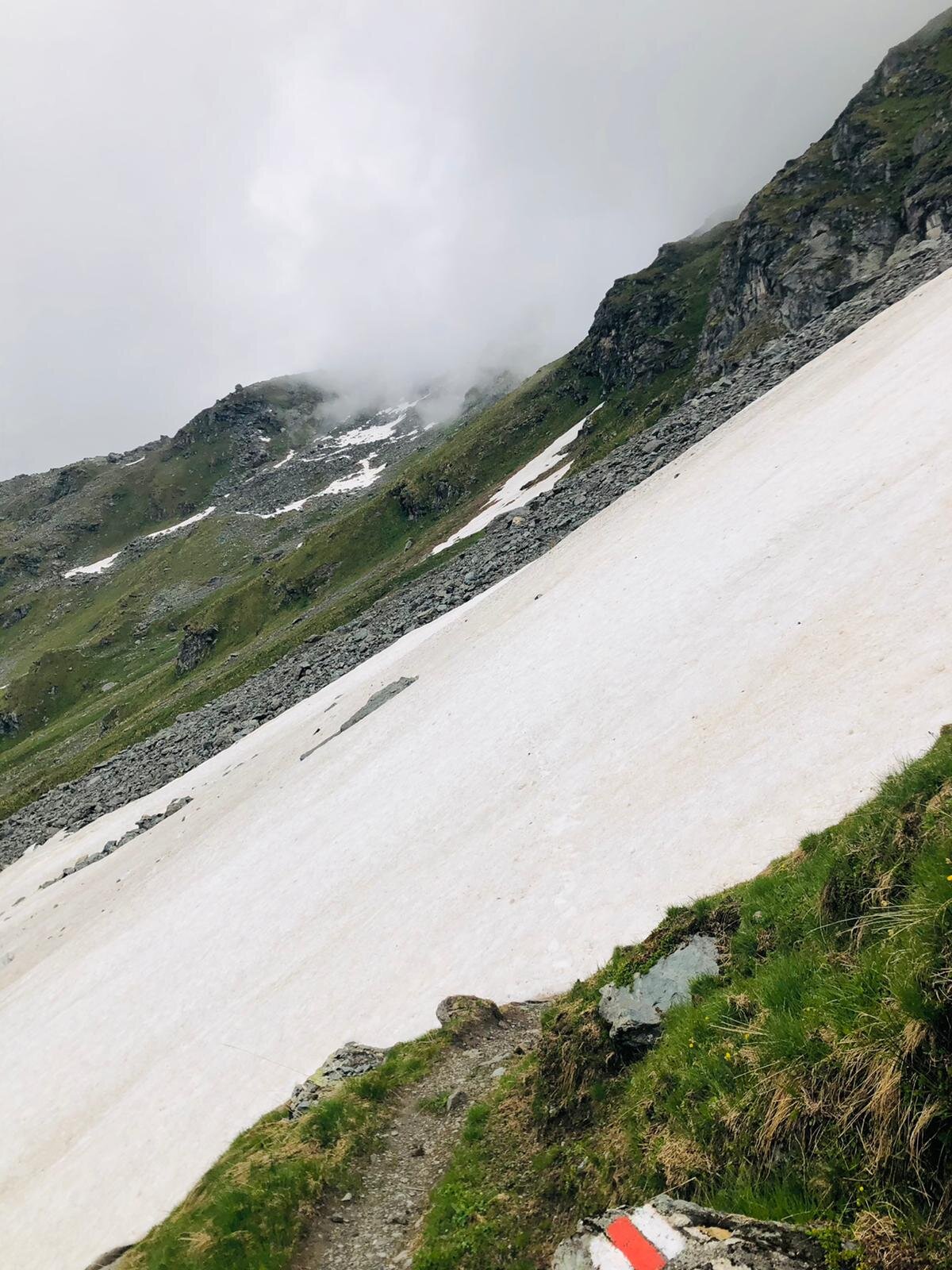This color photograph in portrait orientation captures a rugged mountainside landscape. In the foreground, a path runs diagonally from the bottom left to near the top right, flanked by verdant green and brown grass. At the base, an orange and white striped trail marker sits upon a stone. The terrain transitions into a steep, unblemished expanse of ice or snow, bordered by patches of gray gravel and rock. The hillside slopes upward, showcasing dark, craggy rock faces interspersed with small sections of grass and snow. Above, the sky is heavily overcast and bathed in a misty gray, with dense, fog-like clouds descending almost to ground level. A white cumulus cloud crests the hilltop, adding to the moody atmosphere of this vivid, realistic outdoor scene.